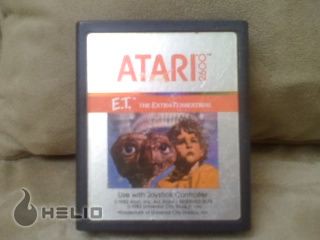This photograph showcases an Atari 2600 video game cartridge for "E.T. the Extra-Terrestrial." The cartridge itself is black with a silver label that features orange and red text. At the top of the label, "Atari" is prominently displayed in red capital letters, followed by an orange banner that reads "E.T. the Extra-Terrestrial" in white text. Below the text, there is a square image of the brown alien E.T. and a young boy gazing upwards to the right. The cartridge is placed on a light brown, tannish-colored couch. In the bottom left corner of the photograph, the word "HELIO" and a flame-shaped symbol—both in a light black color and surrounded by a white border—are visible, possibly as a watermark or logo. The overall appearance is both nostalgic and detailed, emphasizing the iconic elements of this vintage game.